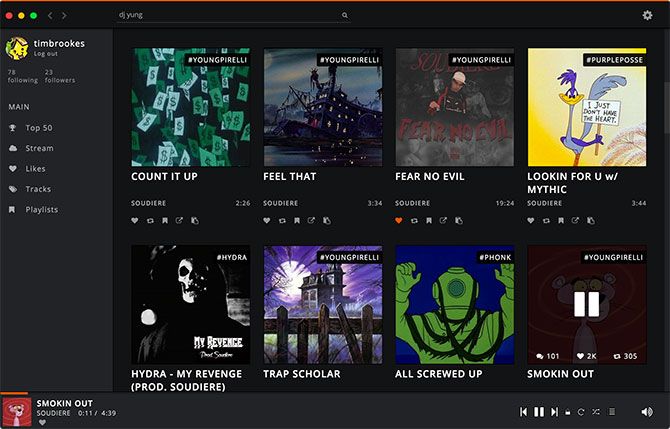The image appears to be a screenshot of a music streaming application on a computer. In the upper left-hand corner, there are three small circles: one red, one yellow, and one green, typical of a Mac OS window interface. Next to these dots are forward and backward navigation buttons, followed by a search bar with the text "DJ YUNG" entered into it. At the far right end of the search bar, there is an hourglass icon in white.

To the extreme right side of the screen, there is a gear (sprocket) icon, usually indicating settings. On the left side, there is an information bar. Here, a circular icon displays a smiling yellow star with eyes, signifying some user interaction or notification. Below this, text reads, "Tim Brooks logged out," and further down lists "78 following" and "23 followers."

This information bar includes multiple sections: "Main" (featuring a trophy icon), "Top 50," "Cloud Stream," "Part Likes," "Ticket Tracks," and a "Banner Playlist." 

Below this, the main content area showcases a grid of album artwork in two rows and four columns. The top row includes:
1. "Count It Up" - album art features dollar bills falling from the sky.
2. "Feel That" - album art depicts a wrecked steamboat in a swamp.
3. "Fear No Evil" - album art shows a man wearing a white hat and black shirt, looking directly at the camera.
4. "Looking For You" - album art displays the Roadrunner holding a sign that reads "I just don't have the heart."

The bottom row contains:
1. "Hydra For My Vengeance" - album art portrays a skeleton wearing a gown.
2. "Trap Scholar" - album art shows a haunted house with a picket fence in the foreground and a moonlit background.
3. "All Screwed Up" - album art features a deep-sea diver covered in algae.
4. "Smoking Out" - album art shows a pause button with the Pink Panther in the background.

At the bottom of the screen, there is a playback control section. It displays the track "Smoking Out" by local artist Pink Panther, showing that it is playing track 11 out of a total of 437. Playback controls include back, pause, forward, skip, and mute buttons on the bottom right.